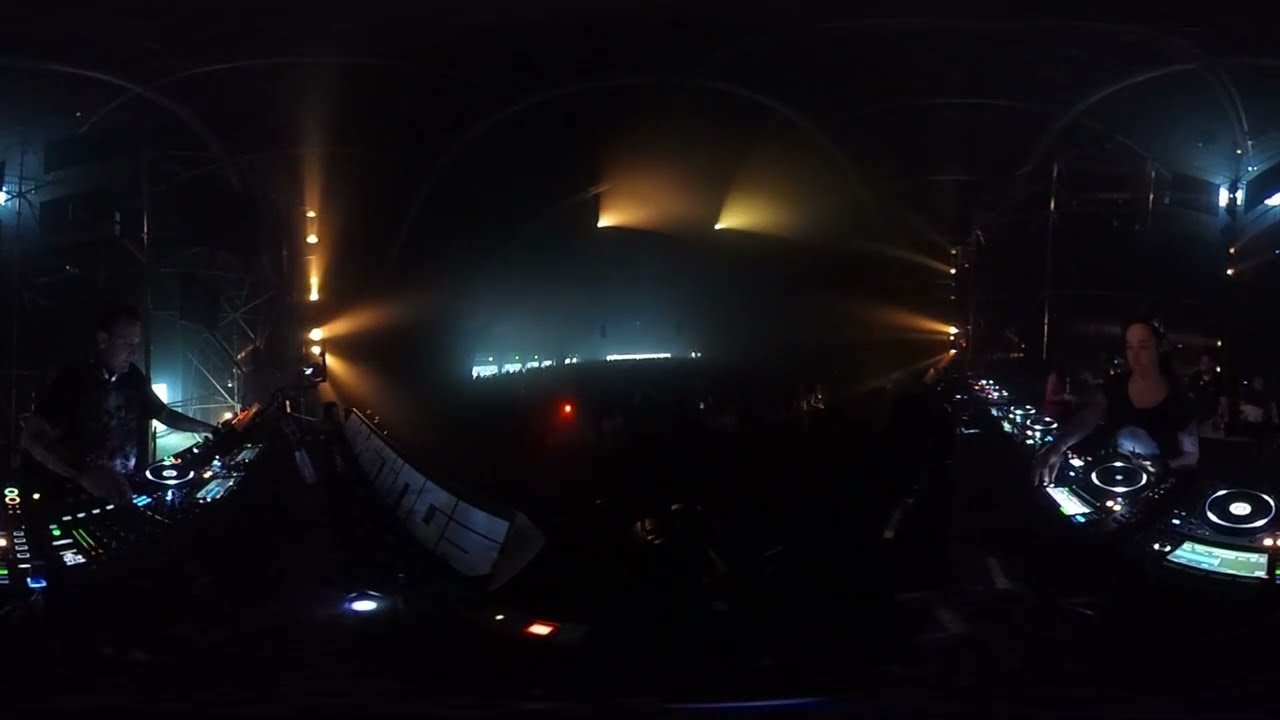The image depicts a dark, immersive DJ event environment featuring two DJs positioned on both the left and right sides of the frame. The left DJ, a male, is intensely focused on maneuvering his audio equipment rife with sliders, buttons, and knobs, bathed in sporadic yellow spotlights illuminating his workspace. The right DJ, a female, operates her equipment surrounded by circular lights, creating a mesmerizing visual effect in the dark setting. Both DJs are dressed in black, blending with the predominantly dark room accented by points of white and yellow light. The middle of the image reveals a pulsating red light, indicating a vibrant crowd gathered at the bottom center. The scene captures the energetic atmosphere of a club or concert where lighting plays a pivotal role in enhancing the auditory experience.